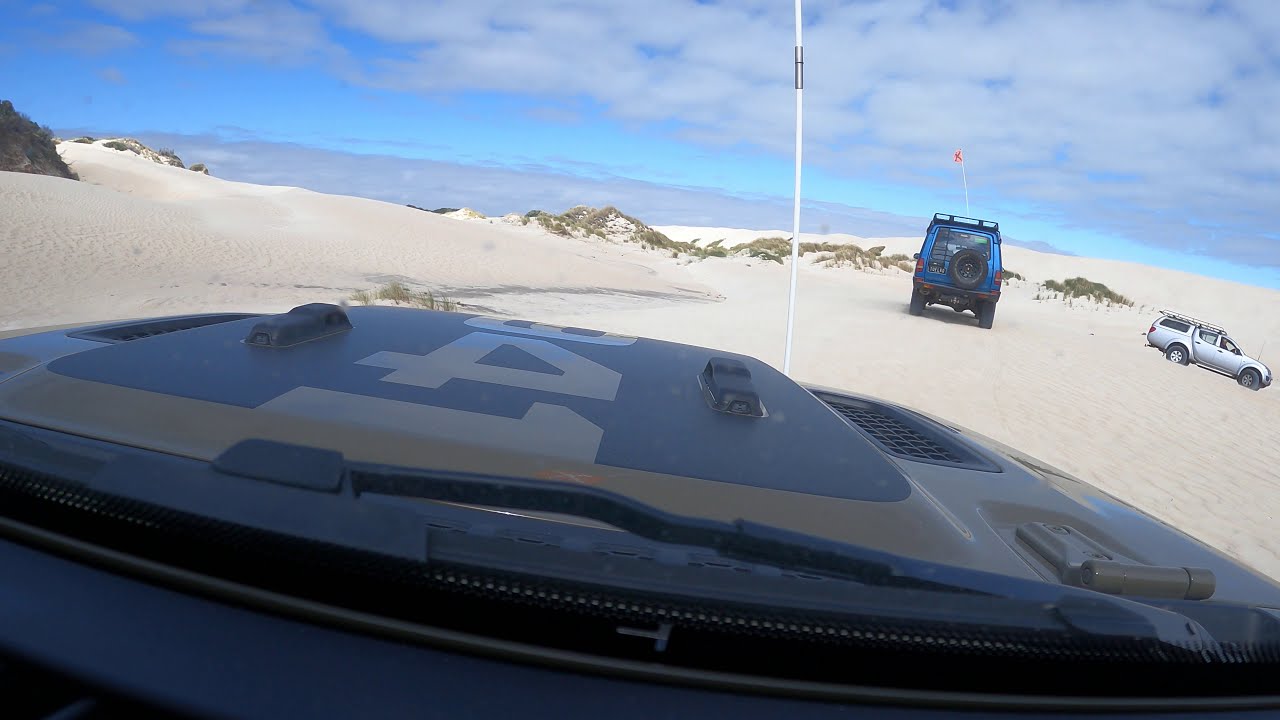In this vivid desert landscape, the image captures an exhilarating off-roading experience under a bright, clear, and sunny sky. The photo is taken from within a rugged vehicle, identifiable by the number "841" painted on its blue roof. Dominating the bottom half of the image, the roof partially obscures the scene ahead, offering a unique perspective from atop a sand dune. Ahead, two other vehicles navigate the challenging terrain: a blue Jeep prominently on the left, carrying a black spare tire and a flag fluttering at the back, and a silver SUV advancing toward the right-hand side. The sky above is scattered with clouds, providing a striking contrast to the expansive sandy landscape below which appears devoid of mountains, emphasizing the vastness of the desert. The geological formations, including scattered rocks, enhance the rugged beauty of the scene, making it an unforgettable adventure in the midday heat.